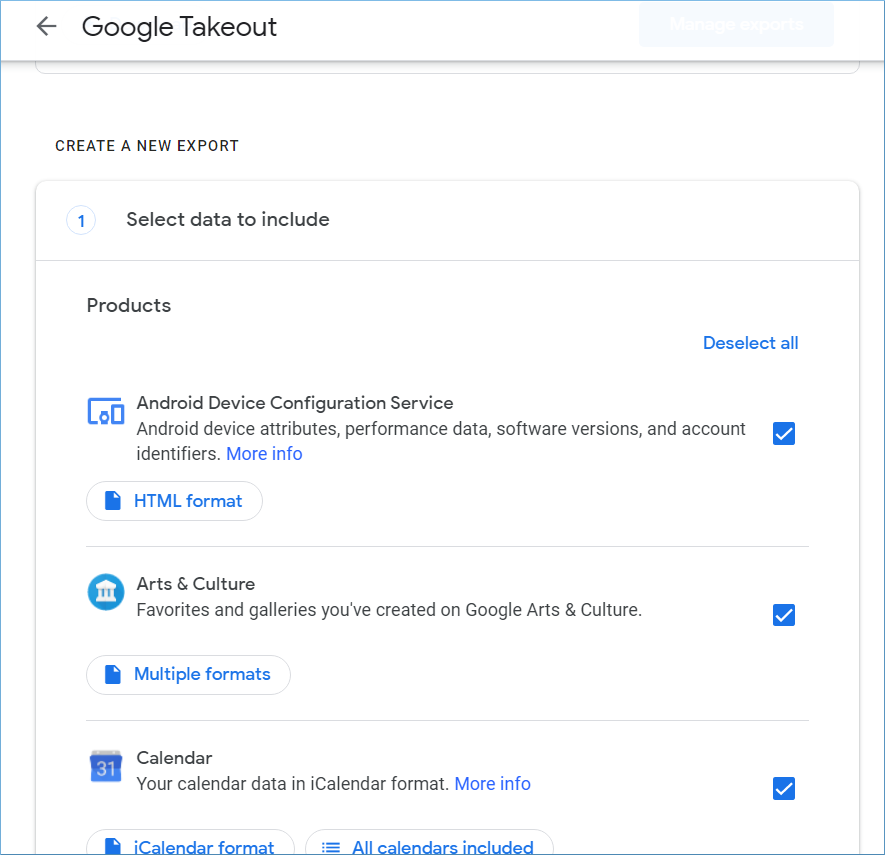The image displays a Google application interface for Google Takeout. At the top, there is a back arrow on the left and the title "Google Takeout." Below that, the section "Create a new export" is highlighted. To the right of this, the option "Select data to include" is indicated in blue.

The interface is set against a white background, with thin gray lines and shadows delineating different sections. 

Scrolling down, the first section is labeled "Products" and includes details like "Android device configuration service," "Android device attributes, performance data," "software versions," and "account identifiers."

The next section, titled "Arts and Culture," lists "Favorites and galleries you've created on Google Arts and Culture." 

Following that, the "Calendar" section mentions "Your calendar data in iCalendar format."

To the right of these section headers, there are square checkboxes, which are highlighted blue with a white checkmark, indicating that all items are selected.

Each section also features an additional button with format options: the first section shows "HTML format," the second section displays "Multiple formats," and the calendar section indicates "iCalendar format" along with the note "all calendars included."